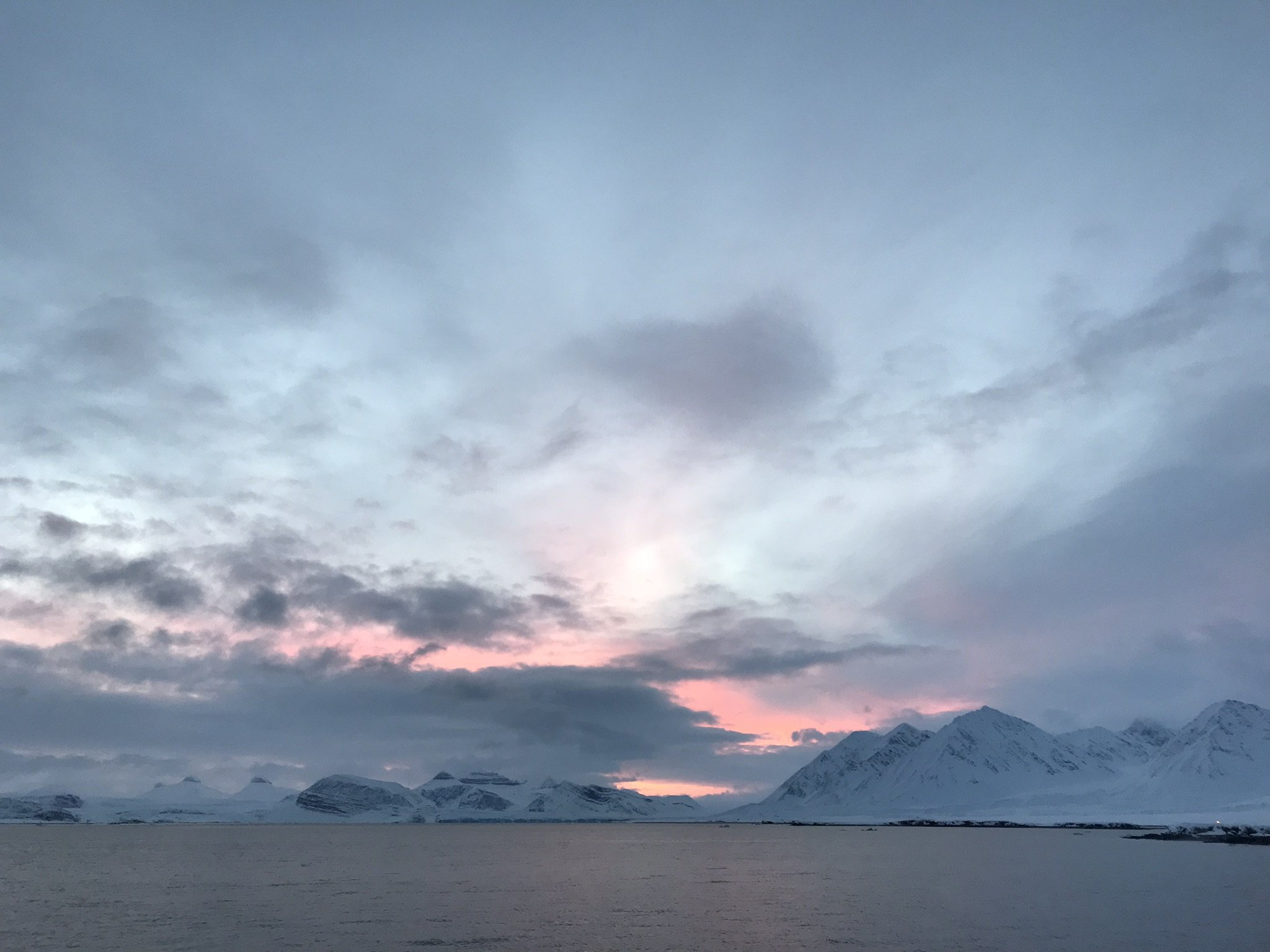This image depicts a serene winter landscape featuring snow-capped mountains against a predominantly cloudy sky. The sky transitions from a lighter blue at the top to a darker hue closer to the horizon, accented with patches of pink and purple, suggesting a low sun. The thick, fluffy clouds appear to be illuminated more towards the bottom, likely by the sun, adding a subtle glow to the scene. Below the sky, the short, white, snow-covered mountains sit in the background, not towering but presenting a formidable, wintry presence. In front of these mountains lies a large lake, its dark, bluish-gray waters mirroring the cold ambiance. The overall atmosphere is one of quiet, cold tranquility, with a distinct chill permeating the scene.